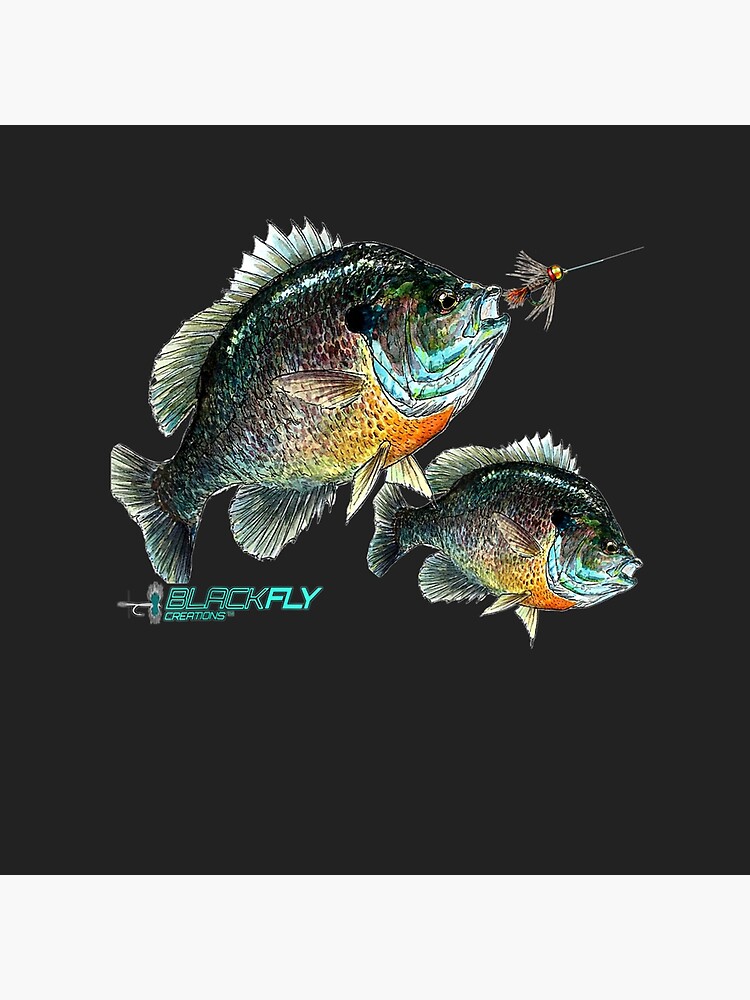This painting, set against a completely black background, features two fish swimming near each other, with intricate detail capturing their vivid colors and textures. The focal fish is angled slightly upward towards the top right corner. It has a dynamic range of colors: a black top, gradient side of light to dark gray, and an underbelly that blends orange and yellow. Its head showcases a stunning array of green, cyan, blue, with dark brown and gray accents. The mouth, slightly open, is hooked by a pink lure adorned with white feathers and a string extending to the right.

The fish's fins are primarily silver, including two small belly fins, a side fin, a dorsal fin, and a tail fin. Bluish hues highlight areas near its mouth and under its chin. Just behind this central fish is a smaller one, similarly colored and positioned, swimming more towards the center right of the image.

In the bottom left corner, "black fly creations" is elegantly inscribed in cyan lettering beside a fish hook. This signature completes the composition, emphasizing the detailed, lifelike representation and the masterful use of color in this captivating artwork.